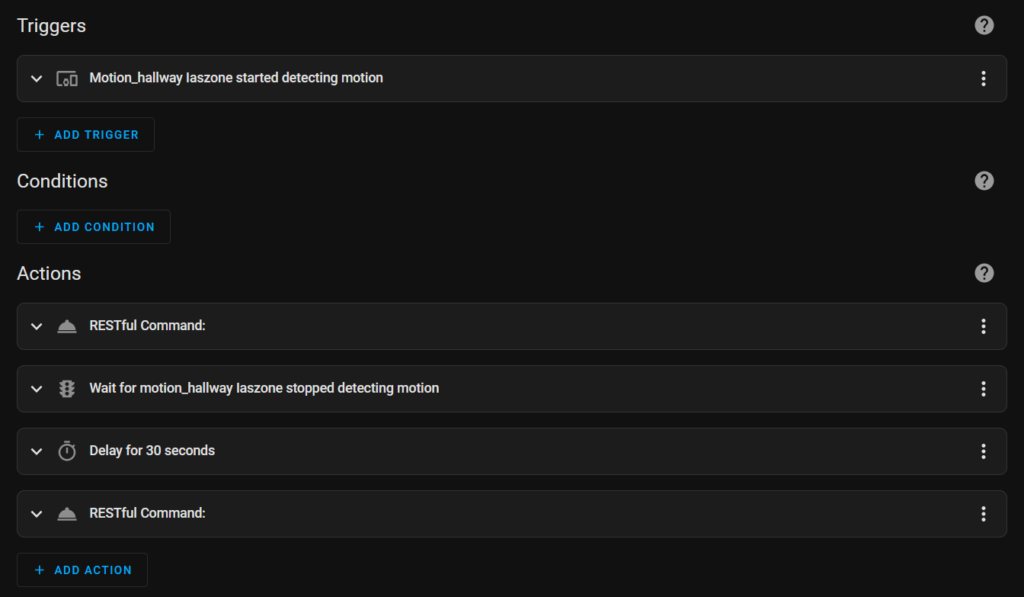The image features a predominantly black background with various segments and elements distinctly highlighted in white and blue text.

In the top left corner, the word "TRIGGERS" is displayed in white letters. Directly below this, a white downward arrow is followed by the words "Motion - Hallway - LAS Zone: Started Detecting Motion."

Beneath this section, a blue plus sign accompanies the text "ADD TRIGGER," both written in blue capital letters.

Proceeding downward, the heading "CONDITIONS" is shown in white letters, with another blue plus sign and the capitalized text "ADD CONDITION" in blue featured just below.

Continuing further down, the section titled "ACTIONS" is also in white letters. This segment is divided into four tabs, each marked with a white downward arrow. The tabs are labeled as follows:
1. "Restful Command"
2. "Wait for Motion - Hallway - LAS Zone: Stop Detecting Motion"
3. "Delay for 30 seconds"
4. "Restful Command"

In the very bottom left corner of the image, there is another blue plus sign accompanied by the capitalized text "ADD ACTION" in blue.

Aligned with the first line, on the far-right side adjacent to the word "TRIGGERS," there is a question mark encircled. Similar encircled question marks are present next to the sections labeled "CONDITIONS" and "ACTIONS," providing consistent visual cues for these segments.

This detailed breakdown of the image captures all textual elements and their specific formatting across the interface.